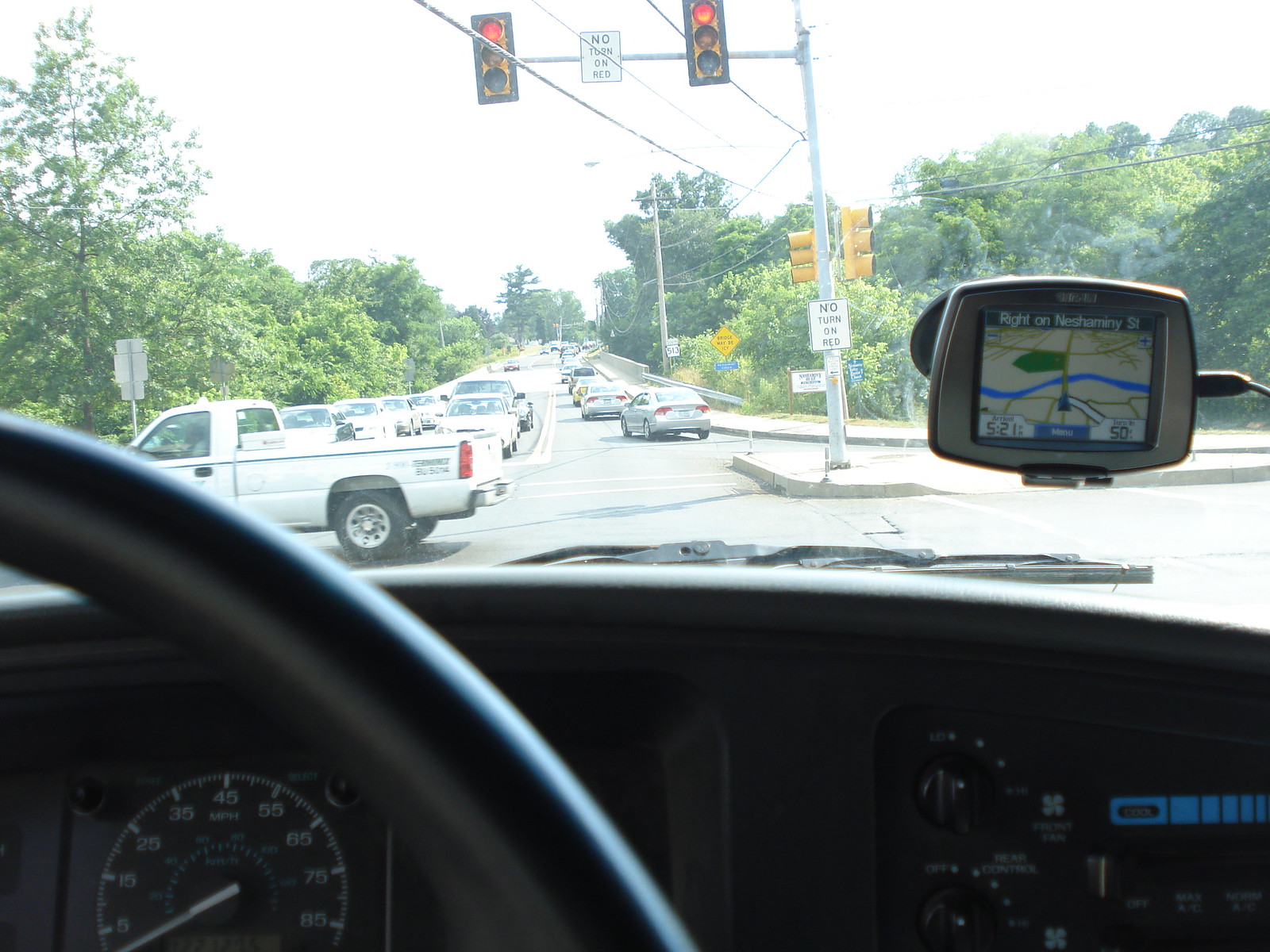This detailed photograph captures the interior of a vehicle that is currently stopped at an intersection, as evidenced by the visible red stoplight. Dominating the foreground, the dashboard, a portion of the instrument panel, and a segment of the steering wheel are clearly seen, along with a clip-on external navigator securely attached to the windshield. The navigator displays a real-time map, which includes the next turn direction, the estimated arrival time, and other navigational information. 

In the background, the intersection buzzes with traffic; vehicles can be seen progressing through the junction and approaching from the opposite side of the street. A prominent feature of the scene is a white truck crossing directly in front of the stationary vehicle, traversing the driver's field of view. The overall scene reflects the activity of a semi-busy street, capturing a moment of urban life from the driver's perspective.